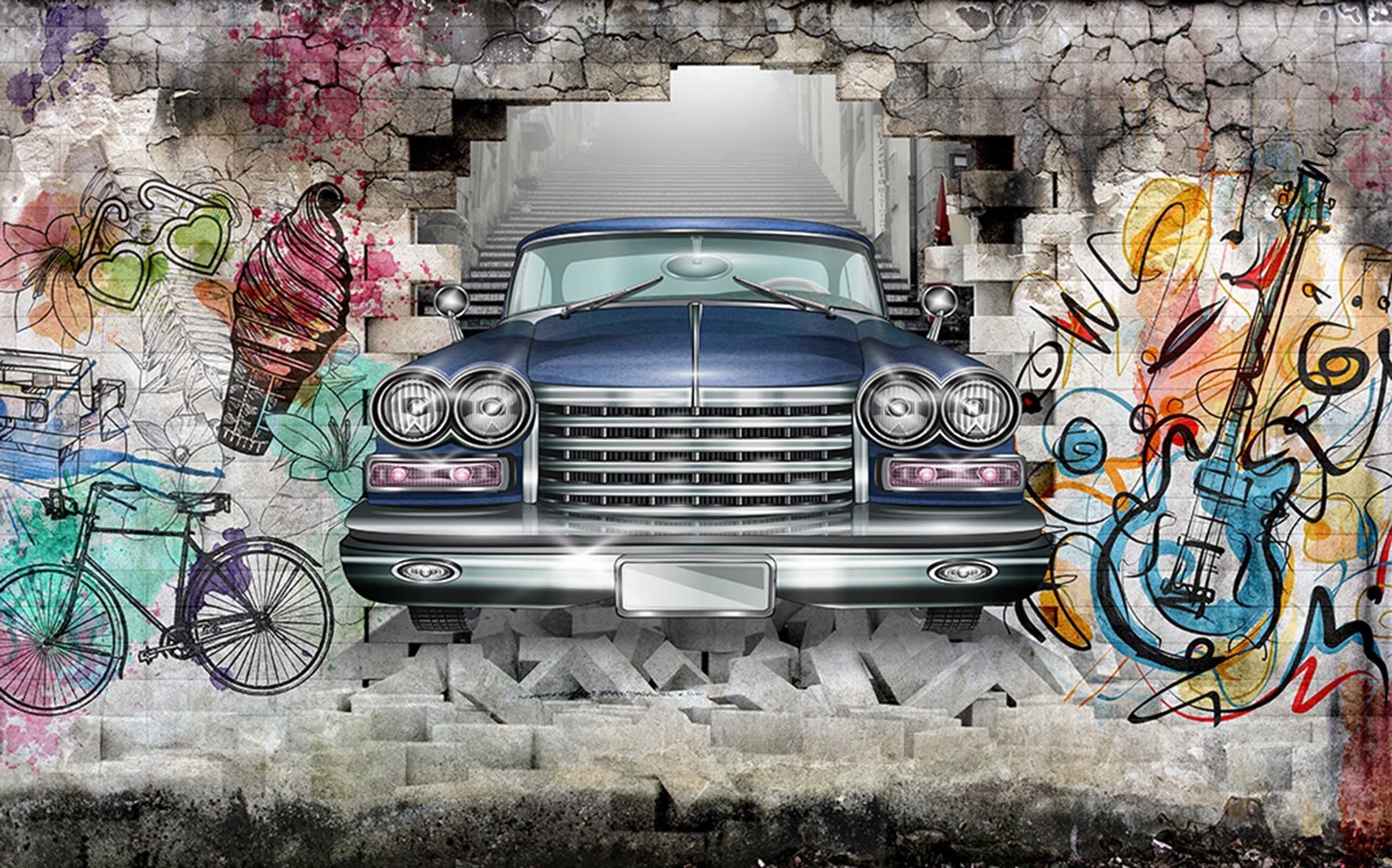This detailed digital illustration showcases a vibrant scene against a brick wall backdrop, adorned with multicolored graffiti reminiscent of a Kandinsky painting. At the center of the image, a large, blue vintage automobile, featuring shiny chrome details, including a grille, bumper, double headlights, and windshield wipers, appears to be bursting through the wall towards the viewer. To the right of the car, a blue and white electric guitar is surrounded by colorful swirls, spots, and lines. On the left side, a soft serve ice cream cone, a pair of heart-shaped sunglasses, lilies, and a 10-speed bicycle are depicted with black line drawings, enhanced with splotches of pink, aqua, purple, red, and orange watercolor for a whimsical effect.